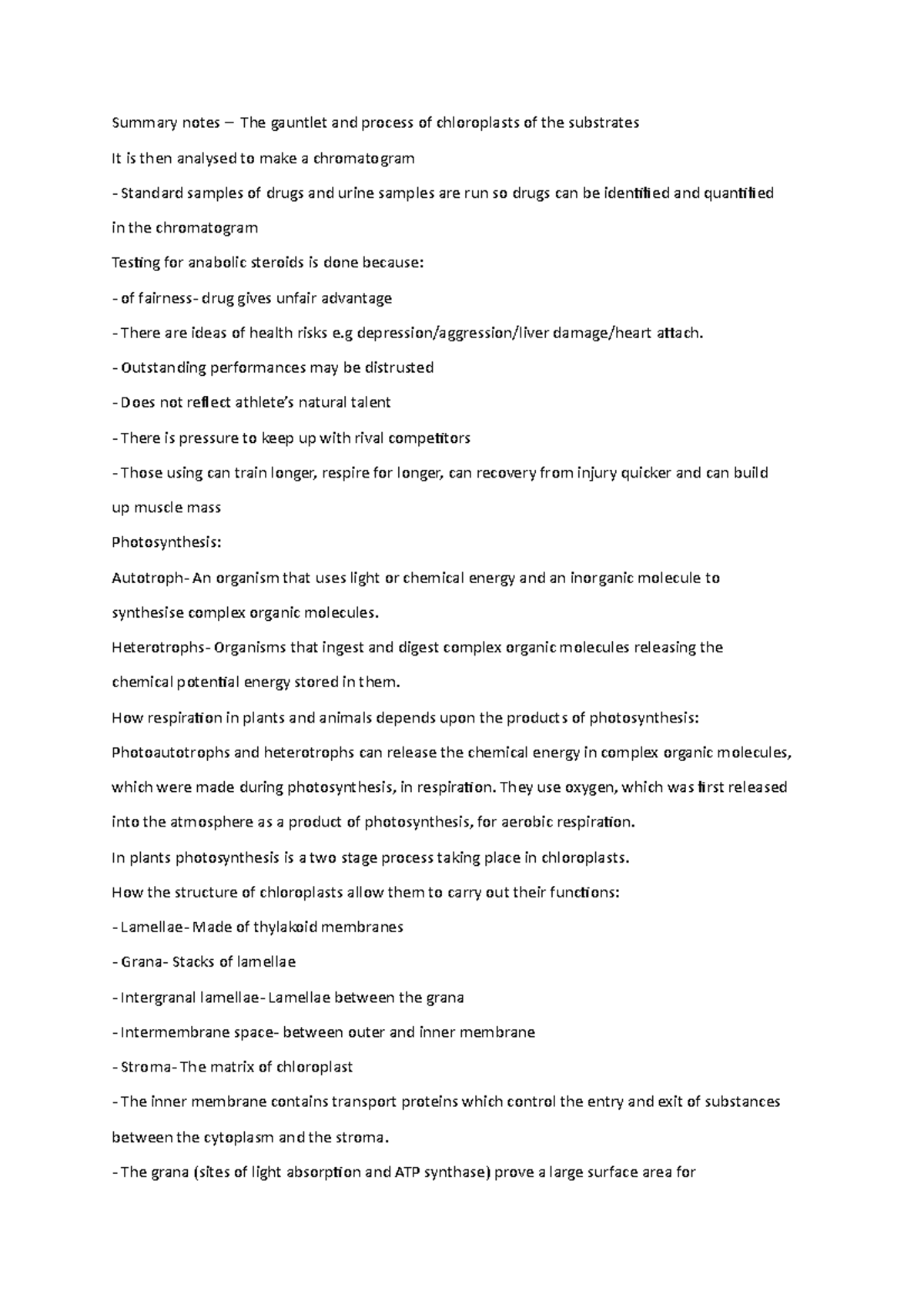This image features meticulously organized summary notes captured on a long, narrow aspect ratio, suggesting they were compiled on a smartphone. At the top, a header reads "Summary Notes," followed by detailed text covering various scientific processes.

The primary section, labeled "The Gauntlet and Process of Chloroplast Substrates," delves into the analysis of substrates through chromatographic methods. Standard procedures for running drug and urine samples are mentioned to identify and quantify drugs within the chromatogram. Notably, it elaborates on the testing for anabolic steroids, listing several points:

- Fairness: Drugs provide an unfair competitive advantage.
- Health Risks: Examples include depression, aggression, liver damage, and heart attack.
- Trust Issues: Exceptional performances raise suspicion, questioning the authenticity of an athlete's natural talent.
- Competitive Pressure: Athletes may resort to drug use to match their rivals' performance.
- Enhanced Training: Drug use enables prolonged training, faster respiration, quicker recovery from injuries, and increased muscle mass.

Another segment focuses on photosynthesis, highlighting fundamental processes and categorizations:
 
- Autotrophs and Heterotrophs: Definitions and distinctions.
- Plant and Animal Respiration: How it relies on photosynthesis outputs.
  
Additional lists pertain to key chloroplast structures and components:
- Lamellae
- Grana
- Integral lamellae
- Intermembrane space
- Stroma

These detailed notes comprehensively encapsulate the intricate processes involved in chloroplast function, steroid testing in sports, and photosynthesis.